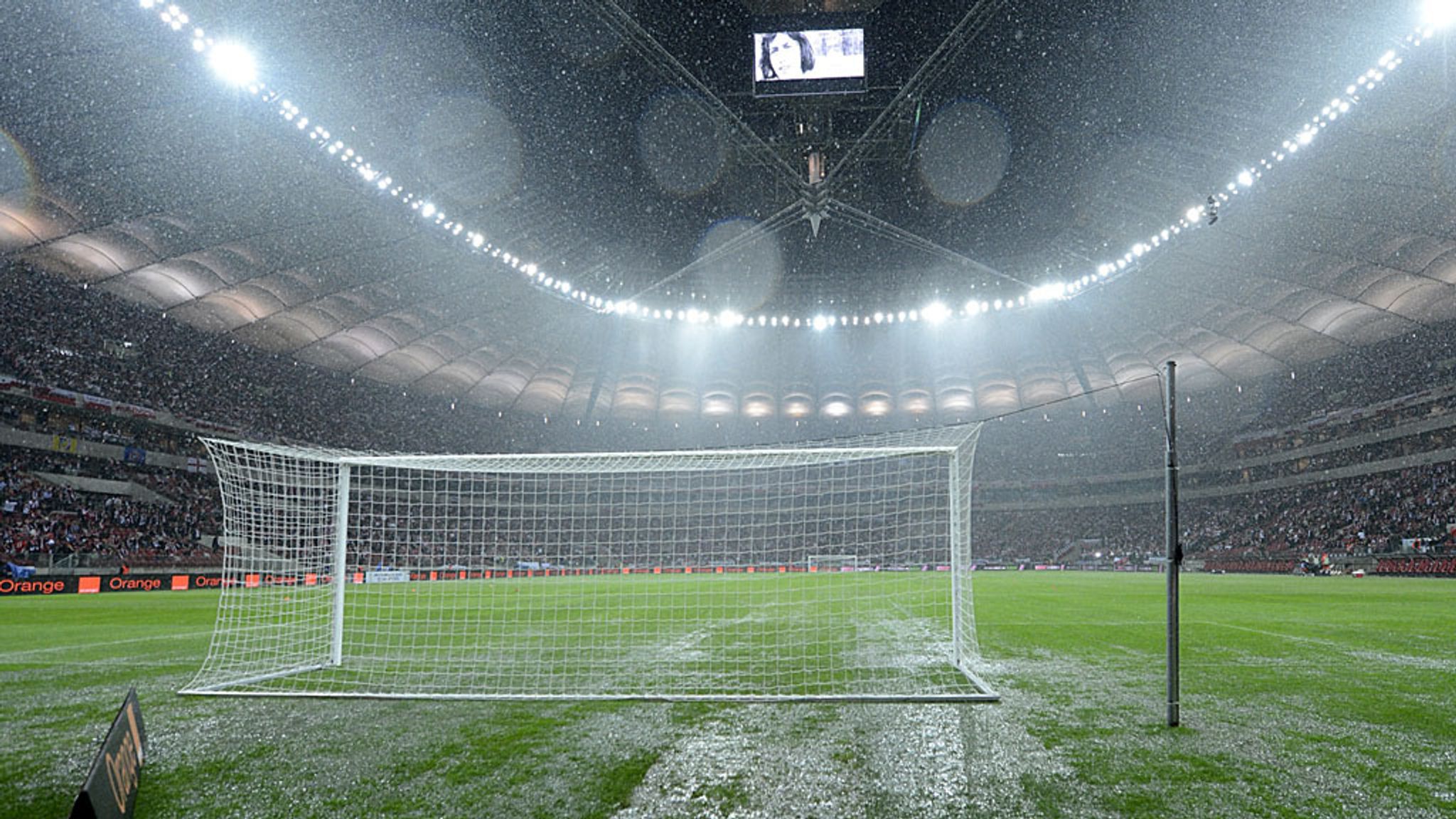The image captures a moment from a packed soccer stadium, viewed from behind one of the goals, focusing on a white frame with a net. Taken from a low vantage point on the grass, the field appears wet with several puddles, suggesting recent or ongoing rain, emphasized by rain specks visible in the air. The brightly lit stadium, featuring a ring of lights around its open or star-speckled ceiling, houses two tiers of seating filled with indistinguishable, tiny spectators. High above, a screen displays an image, possibly a woman's head, and there are advertisements along the side reading "orange." The field itself is empty of players, drawing attention to the glistening grass and a few details such as a metal pole and a small triangular black object on the ground.